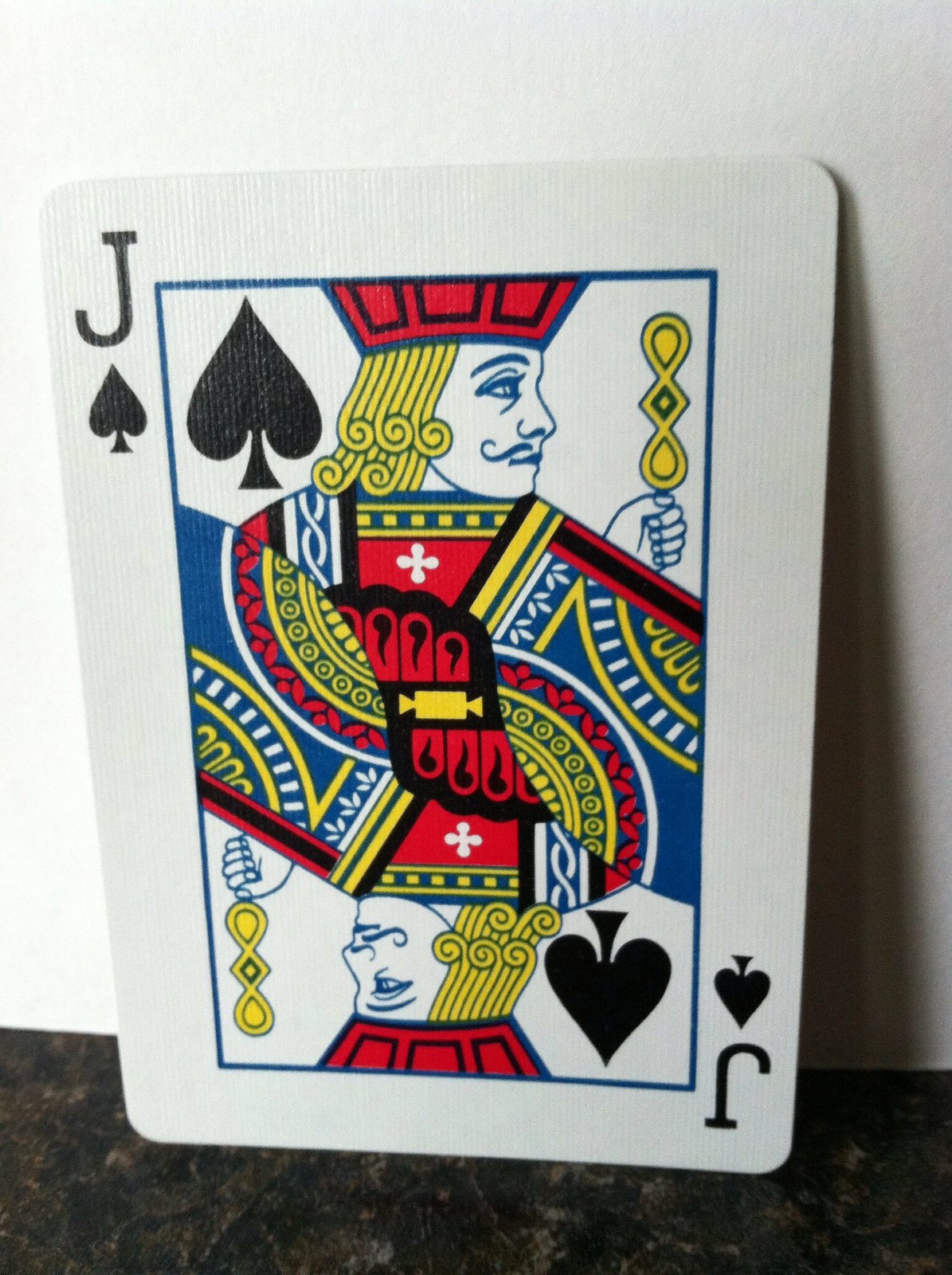This image presents a highly detailed, close-up view of the Jack of Spades playing card. Dominated by rich colors and intricate designs, this black-colored card showcases the letter 'J' in the upper left corner, followed by the distinctive black spade symbol beneath it. Adjacent to these symbols, a vibrant blue rectangle encloses an elaborate depiction of the Jack.

The Jack himself is vividly illustrated, wearing a red crown atop curly yellow hair and a white face accentuated by a curling mustache. His hand grasps a gold, figure-eight-shaped object adorned with a diamond at its center. His attire is a striking combination of gold, red, blue, and white, featuring intricate patterns and details.

Notably, the imagery is mirrored, presenting a double-sided portrait of the Jack. This means that one image of the Jack faces upward while an identical, inverted image faces downward. Central to his costume is a yellow square embellished with two triangles, adding to the elaborate design and overall regal appearance of the card.